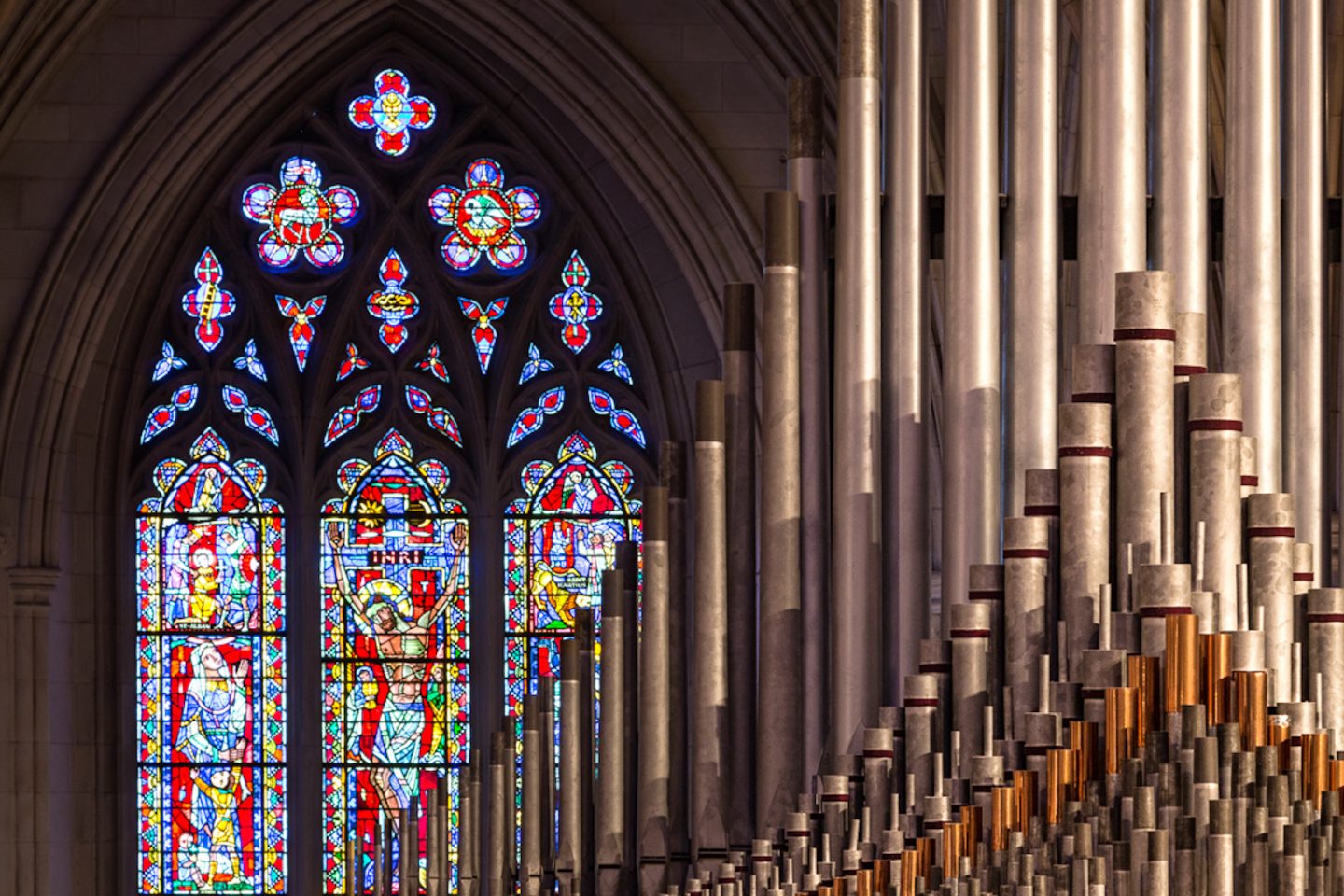This detailed photograph captures the interior of a grand cathedral. Dominating the left side is an expansive arch-shaped stained glass window adorned with an intricate arrangement of floral designs and fleur-de-lis. The vivid colors of red, blue, purple, and yellow bring the window to life, depicting various biblical figures, including a central image of Jesus Christ on the cross. To the left, the Virgin Mary can be discerned, draped in a blue robe, with other saints and disciples adorning the surrounding panes.

Spanning the right side of the photograph, numerous curved, silver metal pipes of a majestic pipe organ rise majestically, punctuated by rows of elegantly tipped gold pipes toward the bottom. These pipes, numbering possibly over a hundred, vary in size and suggest the grandeur of the cathedral's musical instrument. The structure of the cathedral itself is visible in the light gray brickwork, adding a touch of solemnity to this sacred space. Overall, this image beautifully highlights the harmonious blend of artistry and architecture.